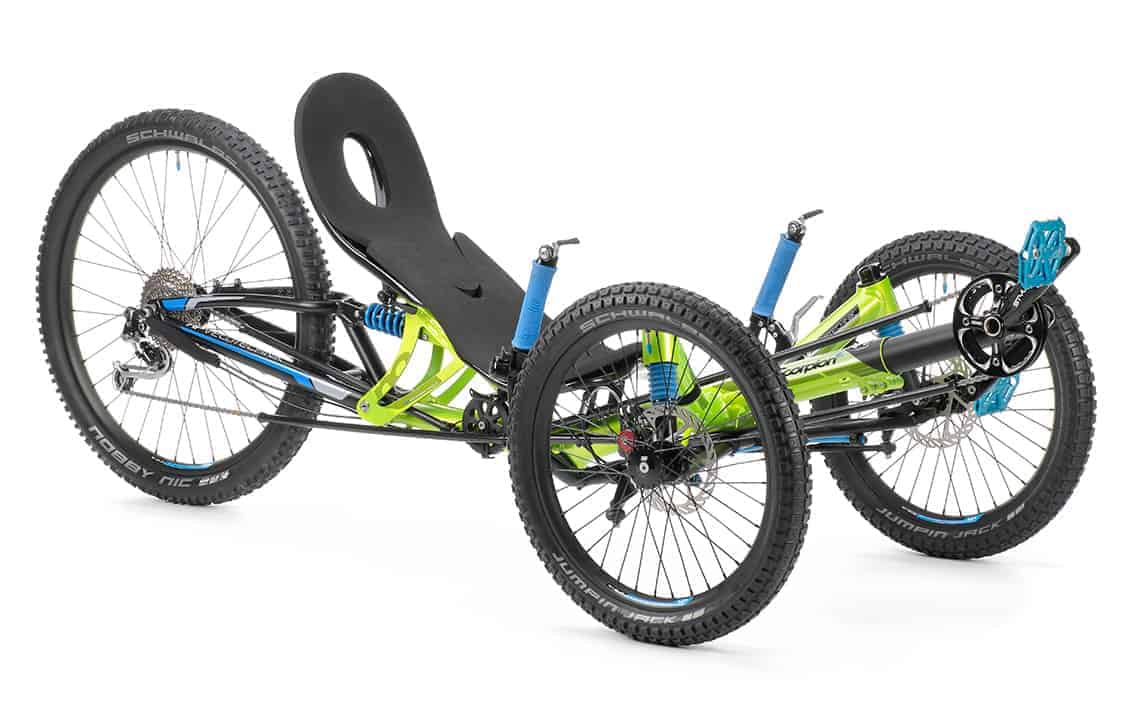The image depicts a distinctive three-wheeled bike known as the Scorpion, featuring a unique reclining seat design. The bike consists of two smaller wheels at the front and one larger wheel at the back. The frame showcases a vibrant combination of blue and neon lime-green colors. The seat is black, possibly made of plastic or foam, with minimal back support and a circular hole in it. Mounted next to the seat are two blue-padded handlebars for arm support, enhancing comfort during rides. The bike is equipped with thick, robust tires for a comfortable riding experience, with the rear wheel branded with "Nobby Nick" text in white. Additionally, the bike includes blue pedals positioned in front. Overall, this riding apparatus, with its comfortable and recumbent layout, appears ideal for leisure cycling and light exercise.